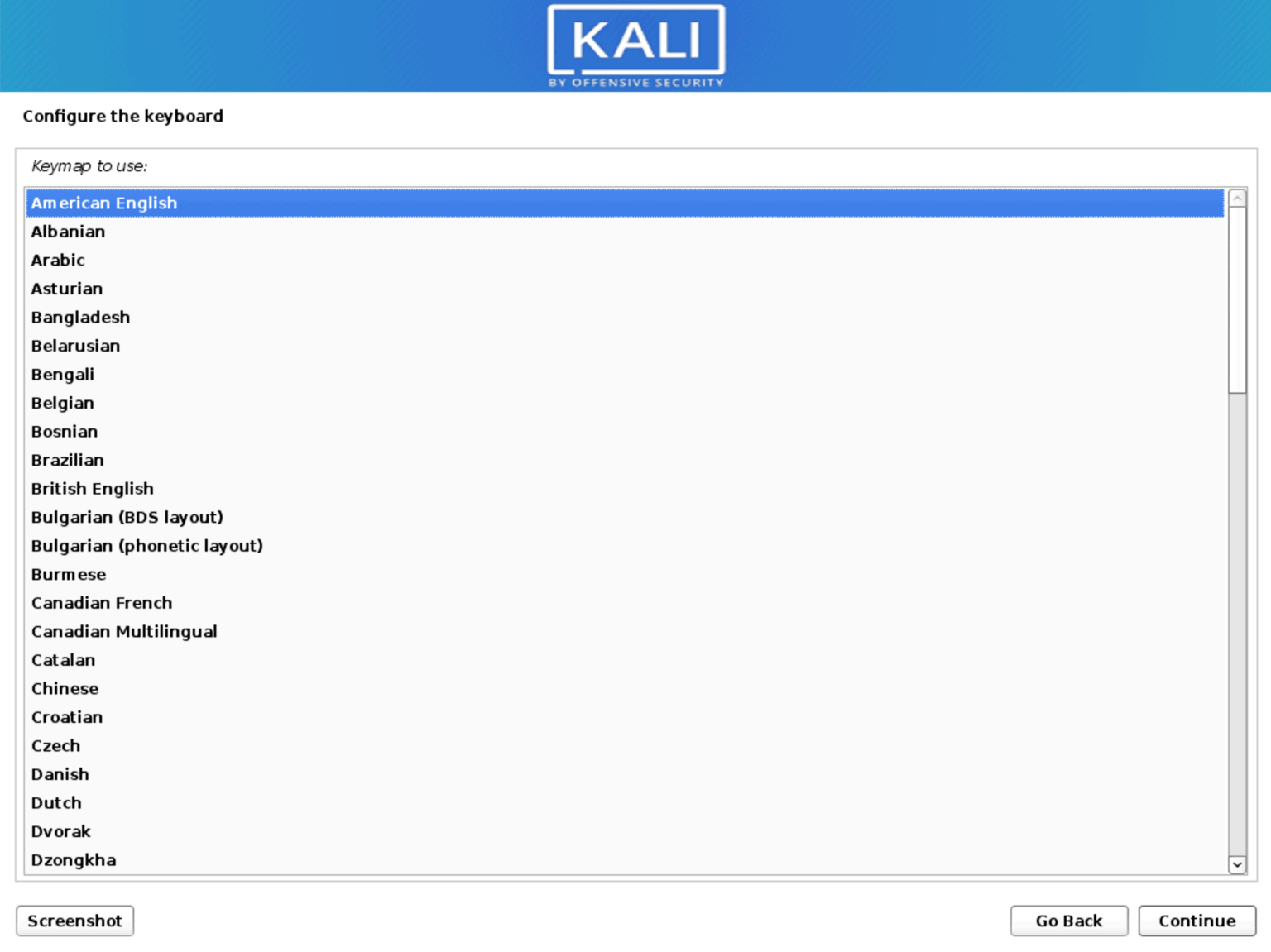The image features a rectangular selection box outlined in white, containing the uppercase letters "K-A-L-I". Below this, in black text, it reads "Configure the Keyboard" followed by "Key Map to Use:". There are numerous language options listed, all in black text, with the topmost option, "American English," highlighted in blue. Subsequent language options include "Albanian, Arabic, Asturian, Bangladesh, Belarusian, Bengal, Belgian, Bosnian, Brazilian, British English, Bulgarian BDS Layout, Bulgarian Phonetic Layout, Burmese, Canadian French, Canadian Multilingual, Catalan, Chinese, Croatian, Czech, Danish, Dutch," and "Dvorak." The last language listed is "Dzongkha." At the bottom of the image, there are three buttons labeled "Screenshot," "Go Back," and "Continue."